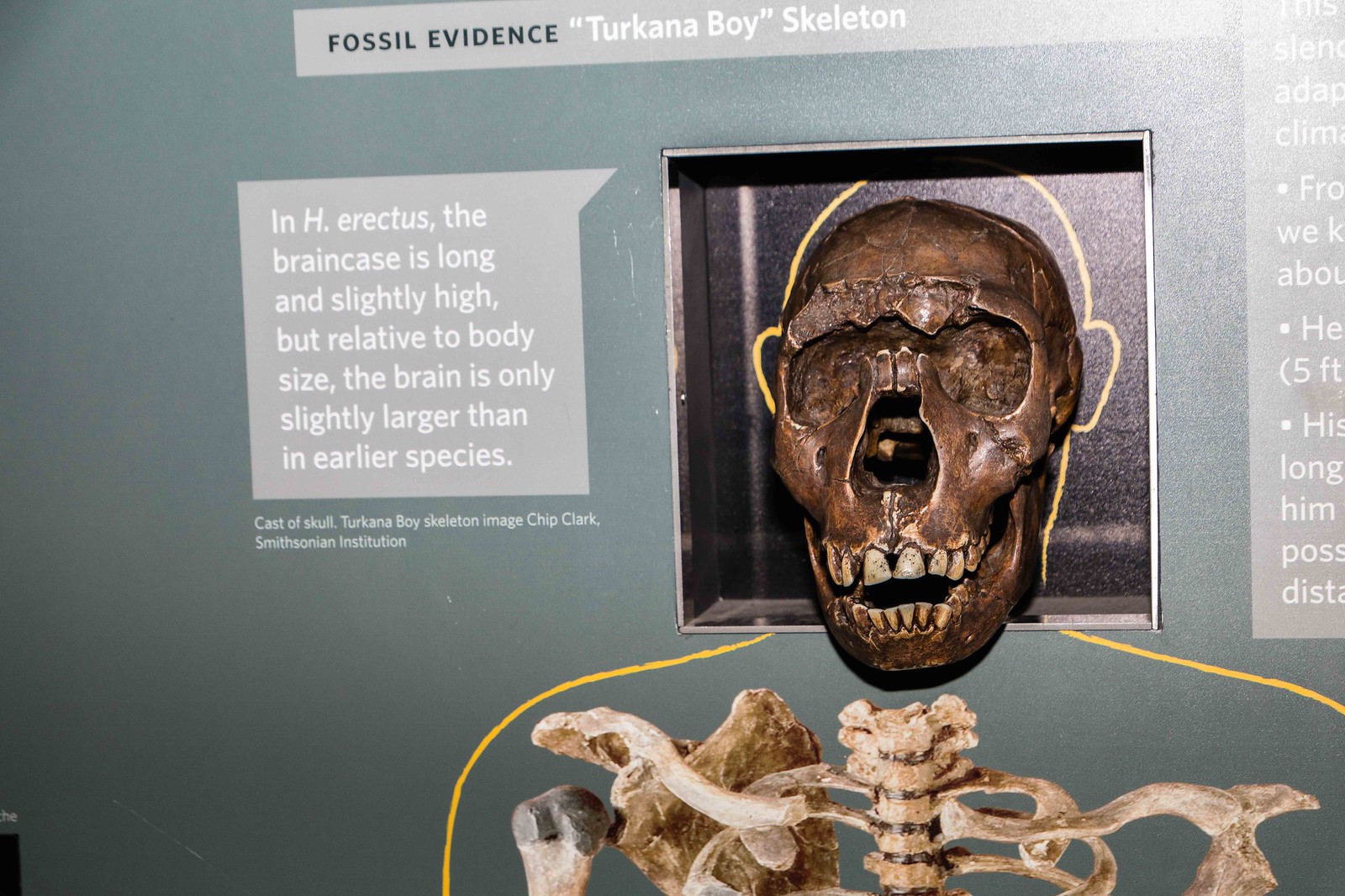The image depicts a museum display showcasing the fossil evidence of the Turkana Boy skeleton. The display features a green wall with a section in a black container housing the actual skull fossil. The text reads "Fossil Evidence of Turkana Boy Skeleton" in uppercase black letters, and it notes that "In H. erectus, the brain case is long and slightly high, but relative to body size, the brain is only slightly larger than in earlier species." Additionally, a cast of the skull is credited to Chip Clark from the Smithsonian Institution. The display also includes a gray rectangle with additional information, as well as an illustration of the rest of the skeleton's bones, although these are not real bones. The skull itself is prominently placed within the green wall, offering a detailed representation of the Turkana Boy's cranial structure.